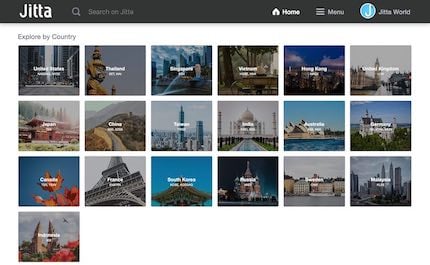The image features a white background with a header at the top that includes a black box displaying the text "JIDA." Below the header, there is a search box, followed by navigation options labeled "Home" and "Menu." Adjacent to these, a blue circle with a white "J" inside is visible, next to the text "JIDA Word." Below these elements, a blue line with small, unreadable text appears.

The main content of the image consists of a series of pictures arranged in a grid format. The grid displays three rows with six images each and a single additional image at the bottom. Each picture is accompanied by white text, though the specifics of the text are not mentioned. The images depict various stunning sceneries, including bridges, oceans, buildings, streets, large statues, and expansive views of water. Notably, landmarks such as the Eiffel Tower and very tall buildings are highlighted, alongside vibrant flowers and picturesque urban landscapes.